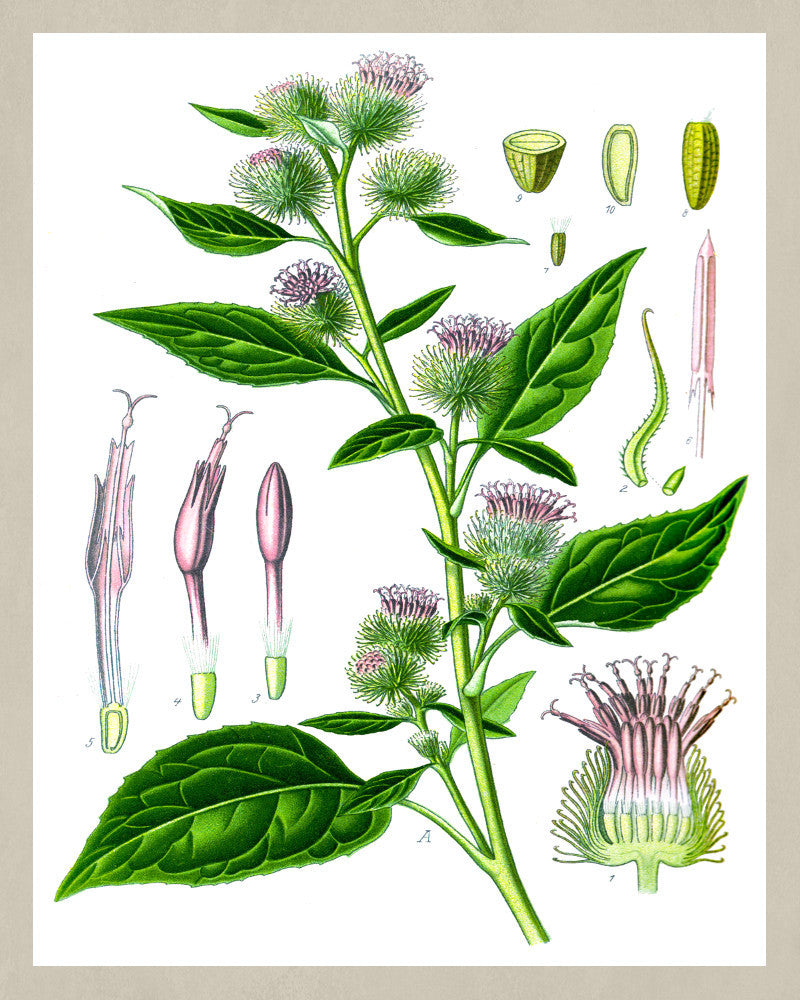This detailed illustration of a thistle bush is presented in a rectangular format, approximately six inches tall and five inches wide, with a light brown, quarter-inch border encasing the white backdrop. The central figure of the drawing features a single long stem adorned with multiple velvety leaves and distinctive purple flowers, each cupped by green tentacles encircling the stamen. These main elements are printed on white paper. The plant is centrally positioned, just right of center at the bottom, extending upwards to just left of center.

On the left side of the main stem, detailed drawings show the transformation of the flower from bud to bloom, labeled sequentially as 3, 4, and 5. Below this, in the lower right corner, a close-up emphasizes the coloration transition from green at the base to white, and finally to purple at the petals. The upper right corner contains additional diagrams depicting various parts of the plant, including what appears to be the seeds. Each stage of the blossom is meticulously illustrated, from a prickly ball to the fully sprouted flower, capturing a total of ten phases. This comprehensive depiction highlights the plant's detailed anatomy and its developmental stages.